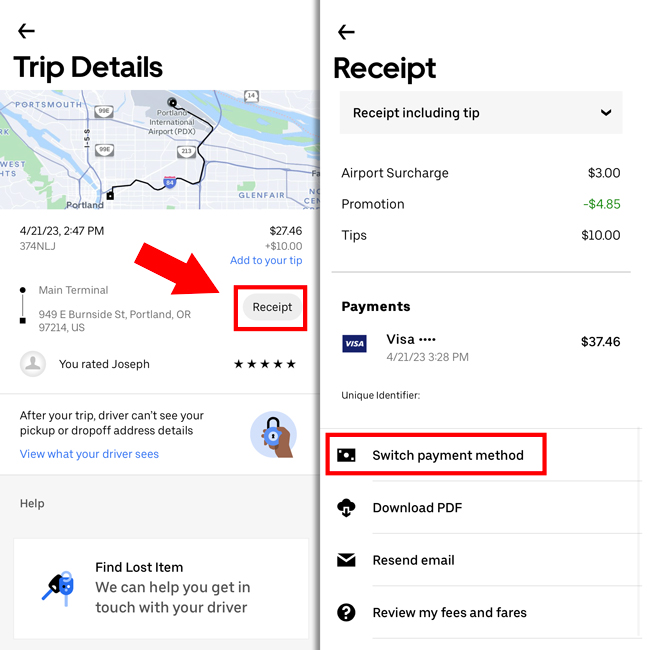The image contains two vertically-aligned screenshots side by side, both in portrait mode.

In the **first screenshot** (left column):
- The upper left-hand corner features a back arrow and bold text reading "Trip Details."
- A map is displayed showing Portland with Route 84 highlighted, leading to the Portland International Airport.
- Beneath the map: "4/21/23, 2:47 PM, $27.46" is listed, followed by "374 NLJ."
- "+$10" is highlighted in blue, indicating the option to "Add to your Tip."
- Below that, it shows "Main Terminal to 949 East Burnside Street, Portland, Oregon."
- On the right, a gray button labeled "Receipt" is highlighted with a red border and a large red arrow pointing to it.
- Beneath this, there's a rating of "Joseph: ★★★★★" and text indicating, "After your tip, the driver can't see your pickup or drop-off address details."
- Links in blue read "View what your driver sees," "Help," and "Find a lost item."

In the **second screenshot** (right column):
- The top has a back arrow and bold text saying "Receipt."
- A gray drop-down menu shows "Receipt including tip."
- Below, charges and discounts are itemized:
  - "Airport surcharge: $3.00"
  - "Airport promotion: -$4.85" (likely a discount)
  - "Tip: $10.00"
- Payment information indicates:
  - "Visa" at "4/21/23, 3:28 PM"
  - Total paid: "$37.46"
- At the bottom, beneath a gray line, "Unique Identifier" information is present with options highlighted in red:
  - "Switch Payment Method"
  - "Download PDF"
  - "Resend Email"
  - "Review my Fees and Fares"

The person who captured these screenshots seems focused on the receipt details, tips, discounts, and payment options.